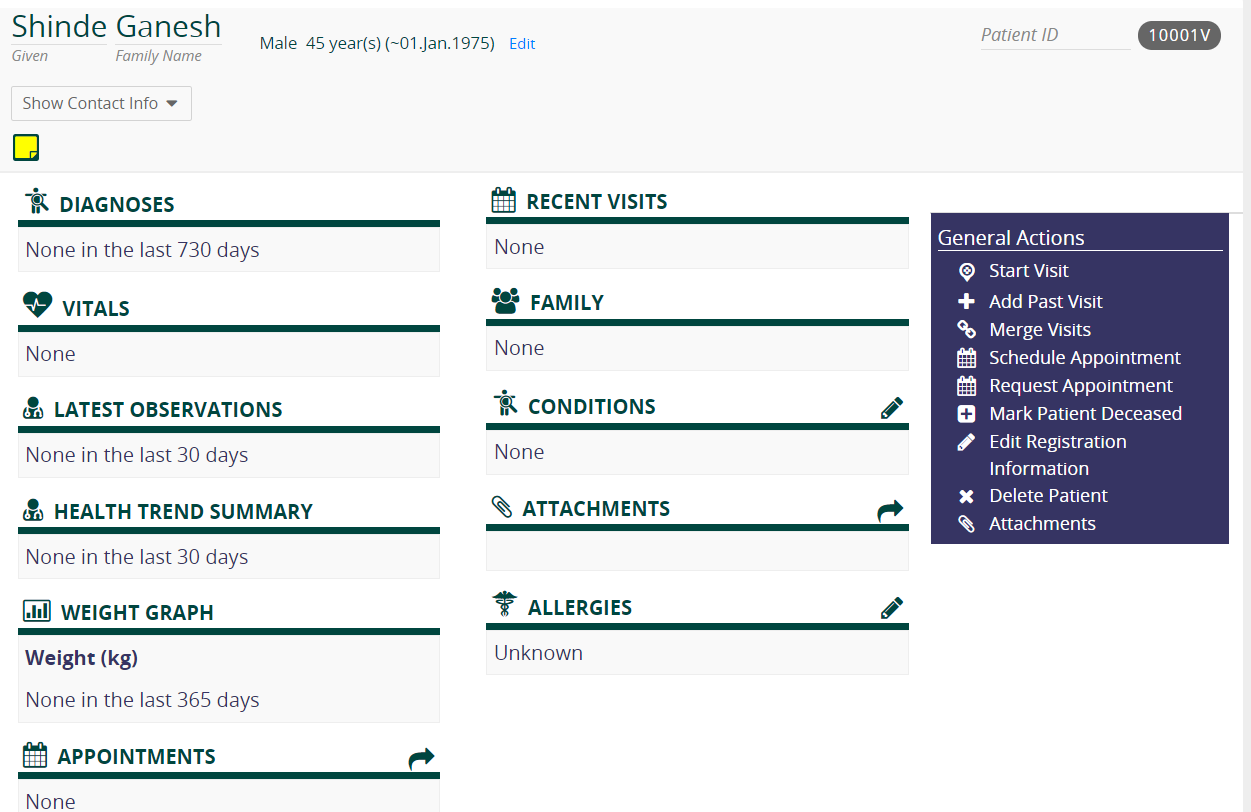This image displays a detailed profile of a male individual named Shind Ganesh. The profile is highlighted in a light gray horizontal bar stretching across the top of the image. 

At the top left corner, "SHIND" is prominently written in black font, followed by the last name "Ganesh." Below his name, it is stated that Ganesh is a 45-year-old male, with his date of birth listed as January 1, 1975. 

On the upper right-hand side of the image, "Patient ID" is labeled, followed by a gray button-like box displaying the ID "10001V."

The lower section of the image is divided into several informational categories:

- **Diagnosis:** No diagnoses recorded in the last 730 days.
- **Vitals:** No vital statistics recorded.
- **Latest Observation:** No observations recorded in the last 30 days.
- **Health Trend Summary:** No trends recorded in the last 30 days.
- **Wake or Activity:** No activity data recorded in the past 365 days.

Overall, the image serves as a comprehensive but currently uneventful medical profile of Shind Ganesh.